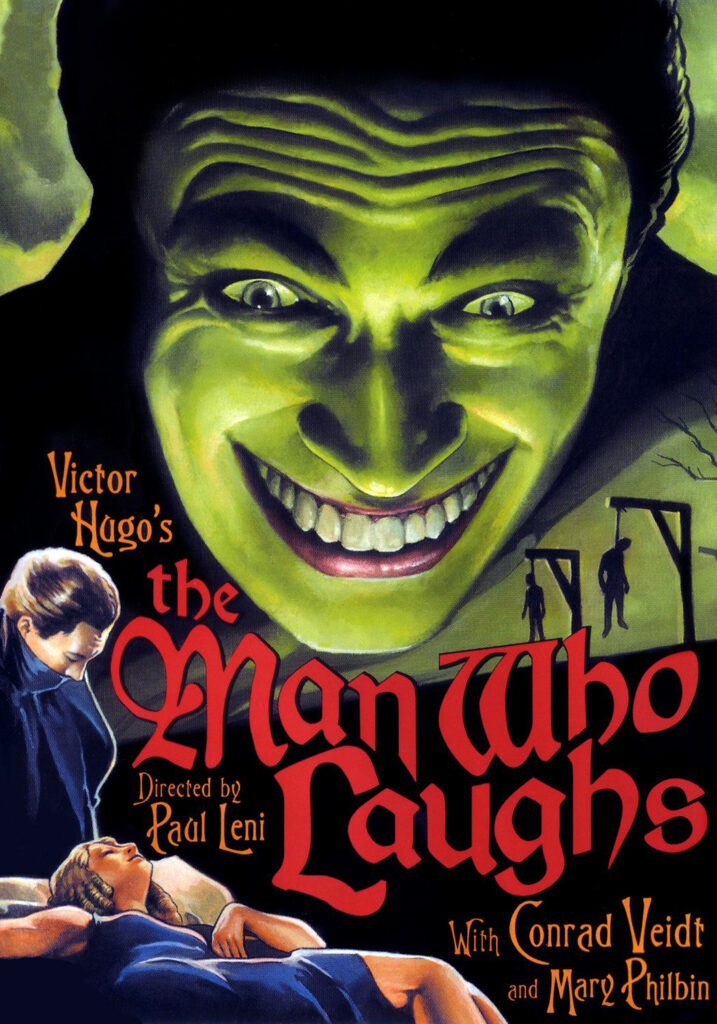This vintage movie poster for the classic film "Victor Hugo's The Man Who Laughs," directed by Paul Leni, prominently features a large, green-tinted male face at the top. The man has a menacing, toothy grin, wide eyes, and a furrowed, crinkled forehead, and is looking downward with dark, slicked-back hair. Below, in the lower left corner, an elderly woman in a blue cloak gazes down at a blonde-haired lady in a blue dress, who lies asleep on a couch, her body draped in a relaxed pose. The right side of the poster depicts two men hanging from nooses on gallows poles in silhouette. In the bottom right corner, the names of the lead actors are displayed: Conrad Veidt and Mary Philbin. The poster’s full, rich colors contribute to its eerie and dramatic effect, capturing the haunting essence of the film.